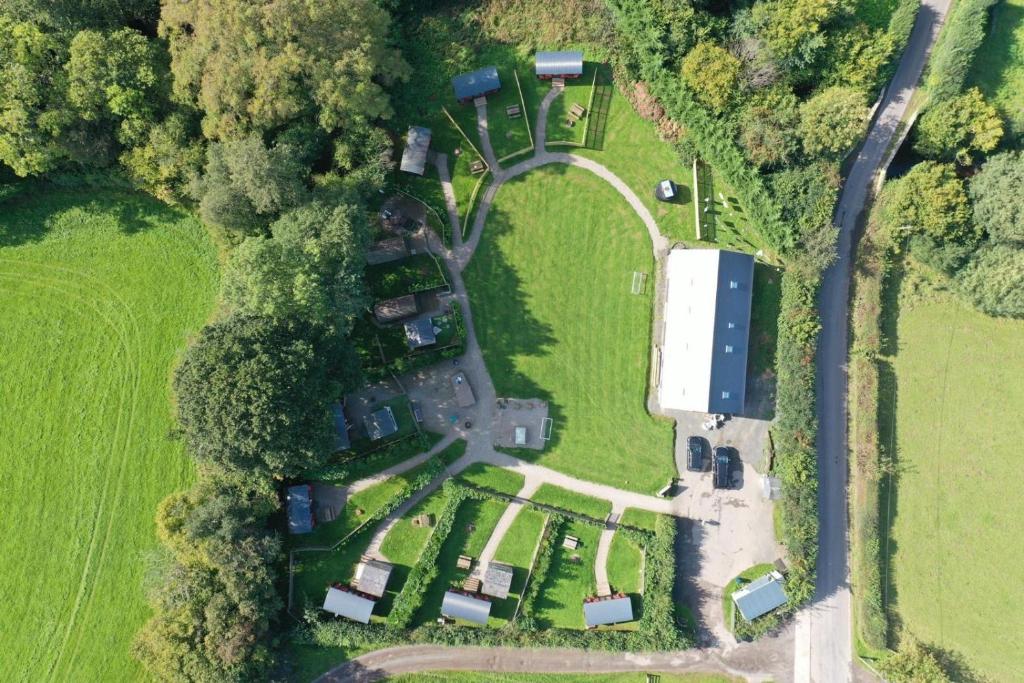The aerial view displays a moderately rural property centered around a large, stark white house with a sloped roof. Surrounding this main structure, there are about six or seven smaller houses, each with distinct blue curved roofs, forming a circular arrangement. These buildings are interconnected by various walkways leading to the main house. In the property's heart lies a lush green patch of grass, free from any structures. To the left and right of the central area, expanses of empty grass and patches of forest merge, enveloping the site in verdant greenery. A road flanks the far right, extending towards the property where two black cars are parked in what resembles a driveway next to the main house. The overall environment appears healthy and well-maintained, with vibrant green foliage accentuating the serene setting.